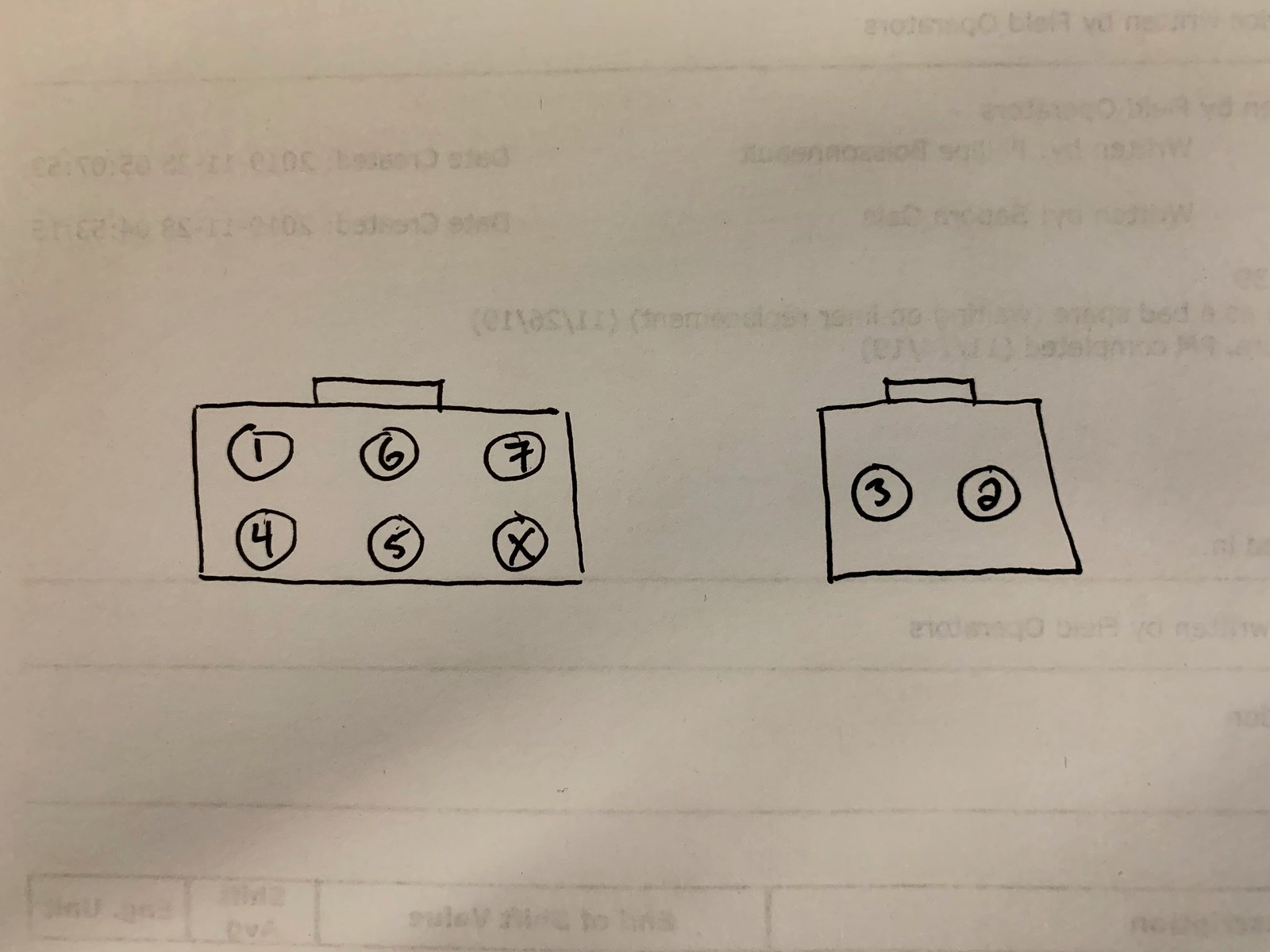The image showcases a drawing on a light gray piece of paper, which appears to have some shading that suggests light is shining on it. Through the paper, typewritten text in black font is faintly visible but unreadable, with some lines and letters appearing in reverse.

At the forefront of the picture, two hand-drawn figures stand out, created using either a marker or a black pen. On the left side of the paper is a large rectangle with a smaller rectangle positioned on top. Inside the larger rectangle, six small circles are arranged, each containing a distinct character: the numbers 1, 6, 7, 4, and 5, and an 'X'.

To the right of this image, aligned parallel to the first box, is a square topped with a small, rectangular pyramid-like box. Within this square are two smaller circles, marked with the numbers 3 and 2, respectively. The meticulous placement and numbering within these shapes suggest an intentional and detailed design.